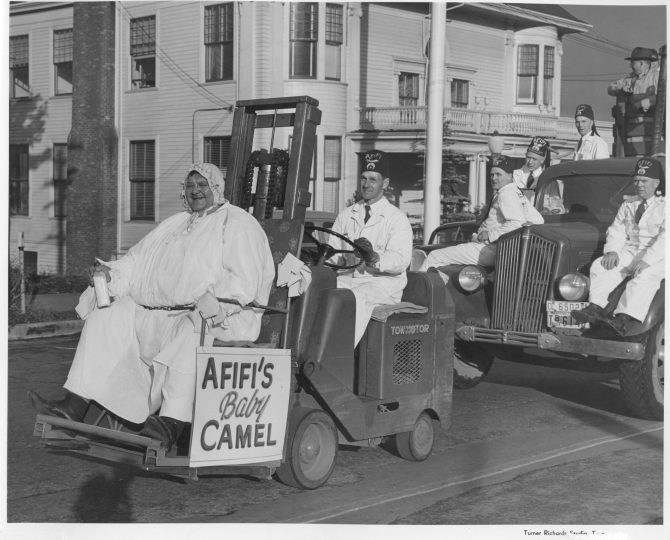This black and white photograph, seemingly from the 1940s to 1960s, captures a lively parade scene transporting a woman on a forklift down a paved street. The woman is seated comfortably in a padded chair with wooden armrests, draped in a white robe with a hood. She is escorted by the Shriners, identifiable by their distinctive tall caps and matching white uniforms. The forklift bears a sign that reads "Afifi's Baby Camel." In the background, a large residential building, possibly a house or apartment, features a second-story balcony, multiple windows, and a brick chimney. An old automobile also appears in the parade, with participants similarly dressed in white attire. The overall scene evokes a sense of yesteryear with its vintage vehicles and classic parade attire.